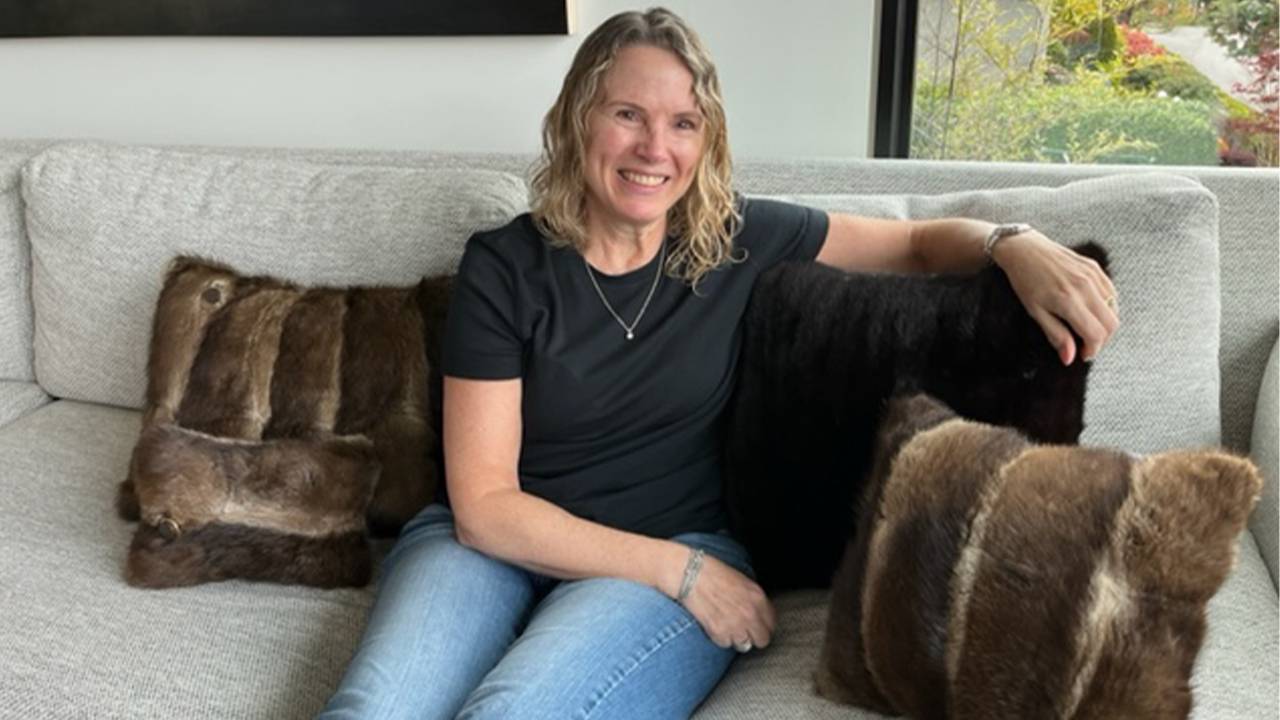In a horizontally rectangular, full-color photograph taken indoors during the daytime, an older blonde woman, likely in her 50s, sits smiling on a light gray, woven cotton couch in a living room. Her shoulder-length hair frames her face as she wears a dark gray heather short-sleeve cotton t-shirt and light blue denim jeans. The living room has a window in the upper right corner showcasing a colorful garden outside, while a black rectangle, possibly the bottom of a TV, appears in the upper left corner. The woman is adorned with a silver watch on her left wrist, a silver bracelet on her right wrist, and a silver necklace with a small circular pendant around her neck. Her left arm is draped over a black throw pillow that resembles fake black hair. She is surrounded by three additional pillows in varying sizes—small, medium, and large—that are brown and appear to be made from imitation deer hair. Her friendly demeanor shines through as she smiles warmly at the camera.